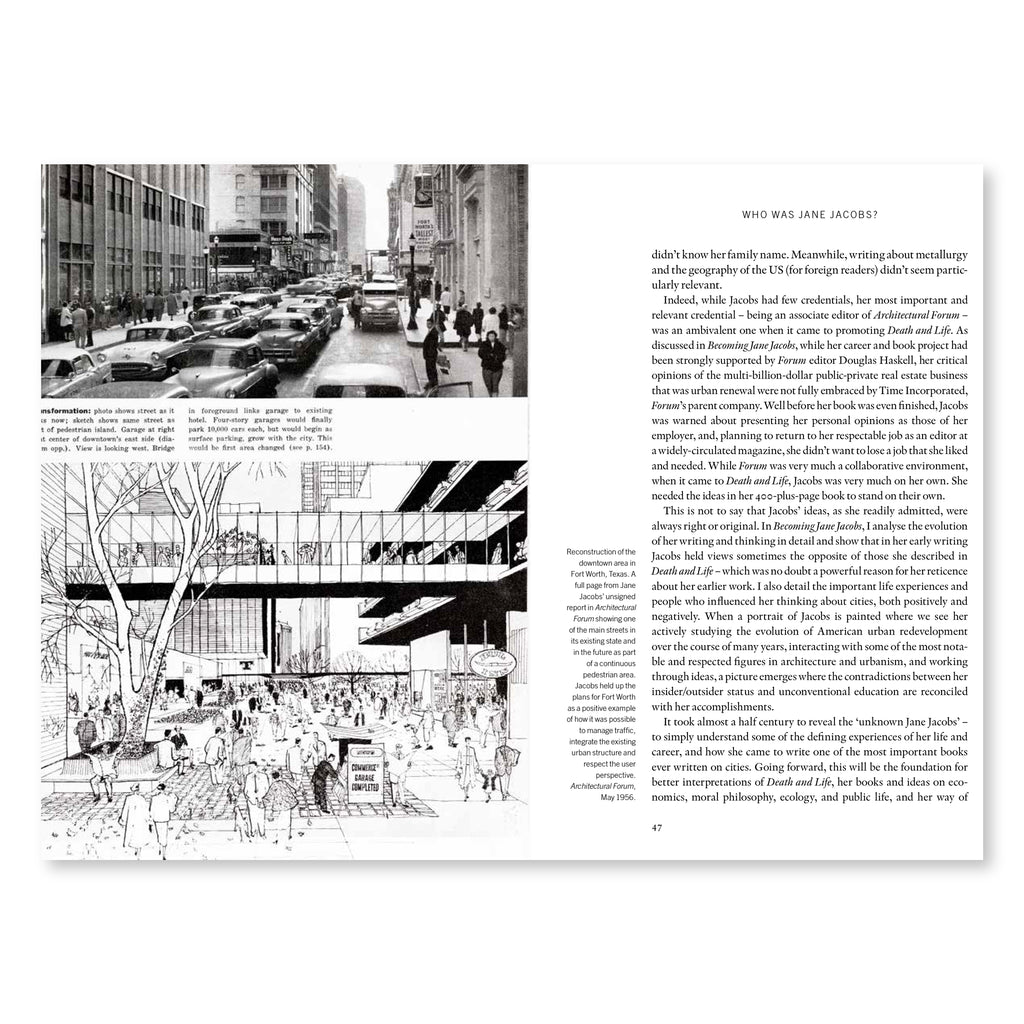A black-and-white spread from a book or magazine features a detailed view that captivates a bygone era. On the right-hand page is the title, "Who was Jane Jacobs?" followed by several paragraphs of text in black typeface on a white background, which is too small to read. The number 47 appears at the bottom of this page. The left-hand page presents a collage of images and illustrations: at the top, a bustling city street from the early 1960s, characterized by antique cars moving towards the viewer and flanked by an array of Manhattan-like buildings. Beneath this photo is a caption, though its text is too small to discern. Below, a cartoon-style pen and ink drawing depicts a busy downtown area with a glass-enclosed walkway bridging two buildings over a courtyard teeming with people enjoying the outdoor space. To the left, a tree emerges from a round planter and arches over the bridge, adding to the intricate urban scene. The overall composition offers a nostalgic glimpse into mid-20th century city life.